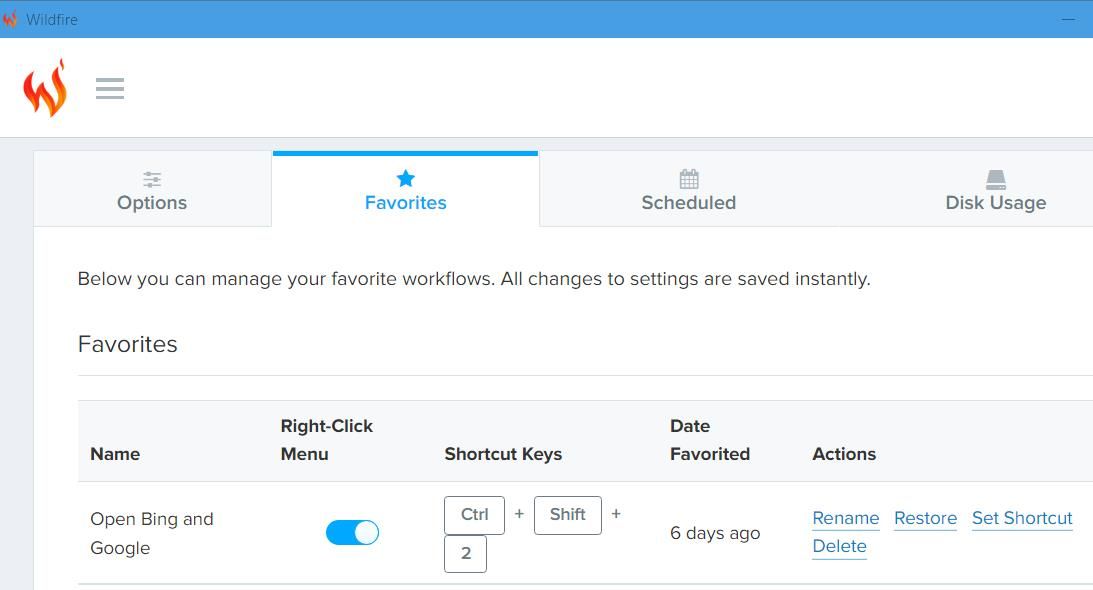The image is a high-quality, detailed screen capture of a software interface. At the top, a thin blue bar highlights the title "Wildfire" in black, accompanied by a yellow and orange flame icon. Directly below this, a menu bar includes a white field containing the flame logo and a series of three gray lines adjacent to it.

The main section features four submenu options, each within a thin gray box: 
1. "Options" with a small line icon,
2. "Favorites" in blue with a star icon,
3. "Scheduled" with a calendar icon,
4. "Disk Usage" displaying a disk icon. 

Beneath these submenus, text in black states: "You can manage your favorite workflows. All changes to settings are saved instantly."

Continuing down, there's a detailed section labeled "Favorites." Here, a specific entry appears in a box that details: 
- **Name**: Open Bing and Google right-click menu
- **Shortcut keys**: Control + Shift + 2 (displayed in a blue box with a white circle)
- **Date favorited**: Six days ago

Under the "Actions" header, there are several blue clickable options: "Rename," "Restore," "Set Shortcut," and "Delete." 

The image is crisp and clear with excellent resolution. The text is bold and dynamic, making it visually appealing and easy to read. The overall layout is clean and well-organized, suitable for easily navigating through the software features.